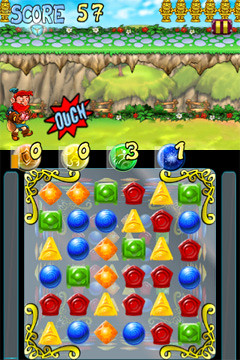This is a vibrant screenshot of a colorful, gem-matching mobile game. The game's background features a bright, contrasting mix of primary colors: a blue sky with white clouds, a grassy terrain with rocks, and a cutaway view of the earth with additional trees. At the top left of the screen, the scoreboard reads "SCORE: 57." To the right is a display of little gold leprechaun depictions, symbolizing lives or game elements, below which lies a pause button. In the middle left section of the screen, a little character resembling a leprechaun with orange-red hair is shown with a starburst exclaiming "ouch." The main gameplay area occupies the lower part of the screen, presenting a grid filled with various vibrant shapes and colors: orange-yellow diamonds, green squares, red house-like shapes, yellow triangles, and blue circles. The game is bordered by an ornate gold frame, and the background features a neutral gray tone, enhancing the colors' brightness and making the overall design vivid and engaging.